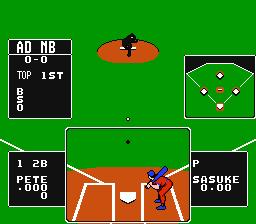The image is a screenshot of an old video game, specifically a vintage baseball game, displayed on a computer screen. The screen has a square aspect ratio, characteristic of older games. The background is a simple solid green, resembling a baseball field. At the top-middle portion of the screen is the pitcher's mound, featuring a small animated pitcher in a throwing stance. 

Towards the bottom of the screen, a larger, zoomed-in section showcases the batter, who is inside a white rectangular box. The batter is positioned on the right side of the box, facing the pitcher, with the home plate clearly visible. The base lines extending from home plate towards the bases can be seen, providing a recognizable layout of a baseball diamond.

On either side of the batter, there are black status squares that display various pieces of information, presumably the game's scoring columns. In the upper left corner of the screen, there's a black area likely used for additional scoring details or game stats. In the upper right corner, an overlay of the playing field is displayed, including the bases, offering an overview of the game's current situation.